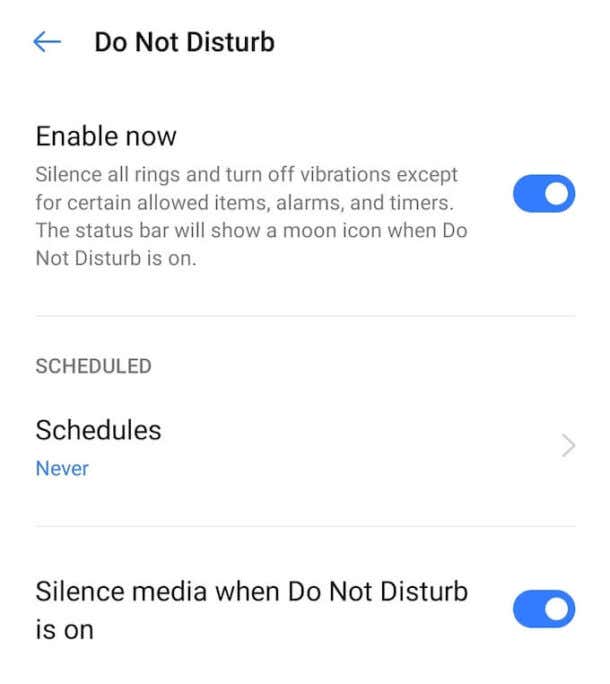The image displays the Do Not Disturb settings on a device, which could be a cell phone or a smartwatch. At the top of the screen, "Do Not Disturb" is prominently written in black letters, accompanied by a blue back arrow, indicating a navigation option to return to the previous menu. Directly below, the option "Enable Now" appears in black text, followed by a description in smaller black letters: "Silence All Rings and Turn All Vibrations Except for Certain Allowed Items, Alarms, and Timers." 

A moon icon is displayed in the status bar when Do Not Disturb is activated, with the toggle switch turned on and highlighted in blue, indicating that the feature is currently enabled. The menu continues with the following options listed in black text: "Scheduled," "Schedules," and "Never." The word "Never" is highlighted in blue, along with an arrow to its right, suggesting further settings or modifications can be made.

Additionally, there is an option labeled "Silence Media when Do Not Disturb is on," written in black text. This feature also has a blue toggle button next to it, set to the on position. The overall design of the settings menu features a simple and clean color scheme: a white background, black text, and blue accents for toggle switches, the word "Never," and navigation arrows.